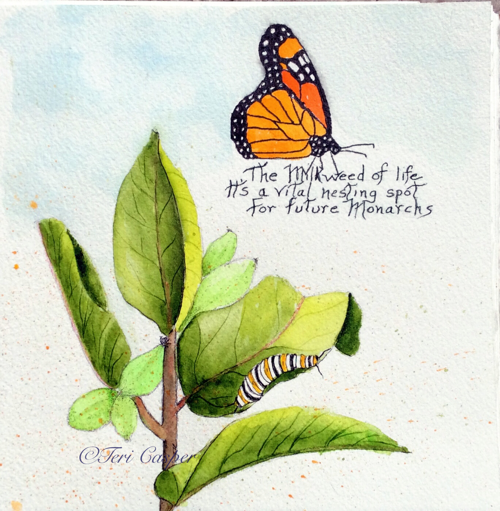This artwork is a delicate, watercolor-like illustration on textured paper featuring the life stages of a monarch butterfly. The background transitions from light blue at the top to white towards the bottom, providing a serene backdrop. In the upper right, a striking monarch butterfly with vibrant orange and black wings, adorned with white dots, hovers gracefully. Below, to the left, a milkweed plant with four prominent leaves and several smaller ones emerges, detailed with a brown vein. A caterpillar, banded in black, yellow, and white, clings to one of the leaves, representing the butterfly's larval stage. The piece is titled "The Milkweed of Life: A Vital Nesting Spot for Future Monarchs," written in elegant black text just below the butterfly. The bottom left corner bears the signature of the artist, Terry Gasper, in cursive, adding a personal touch to this captivating depiction of nature's cycle.